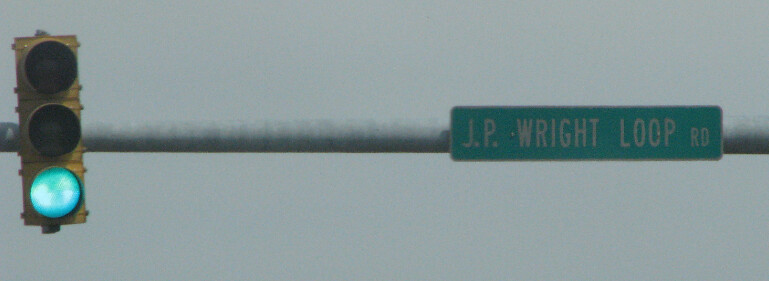The image features a straightforward composition with a light gray background. Horizontally bisecting the photograph is a utilitarian pipe. On the left side of this pipe, there is a yellow traffic light with three vertically-aligned circles; the top two are unlit and black, while the bottom one is illuminated in green. Positioned slightly past the center of the image is a green sign with a thin white border that reads "J.P.WRIGHT LOOP RD" in all capital letters.